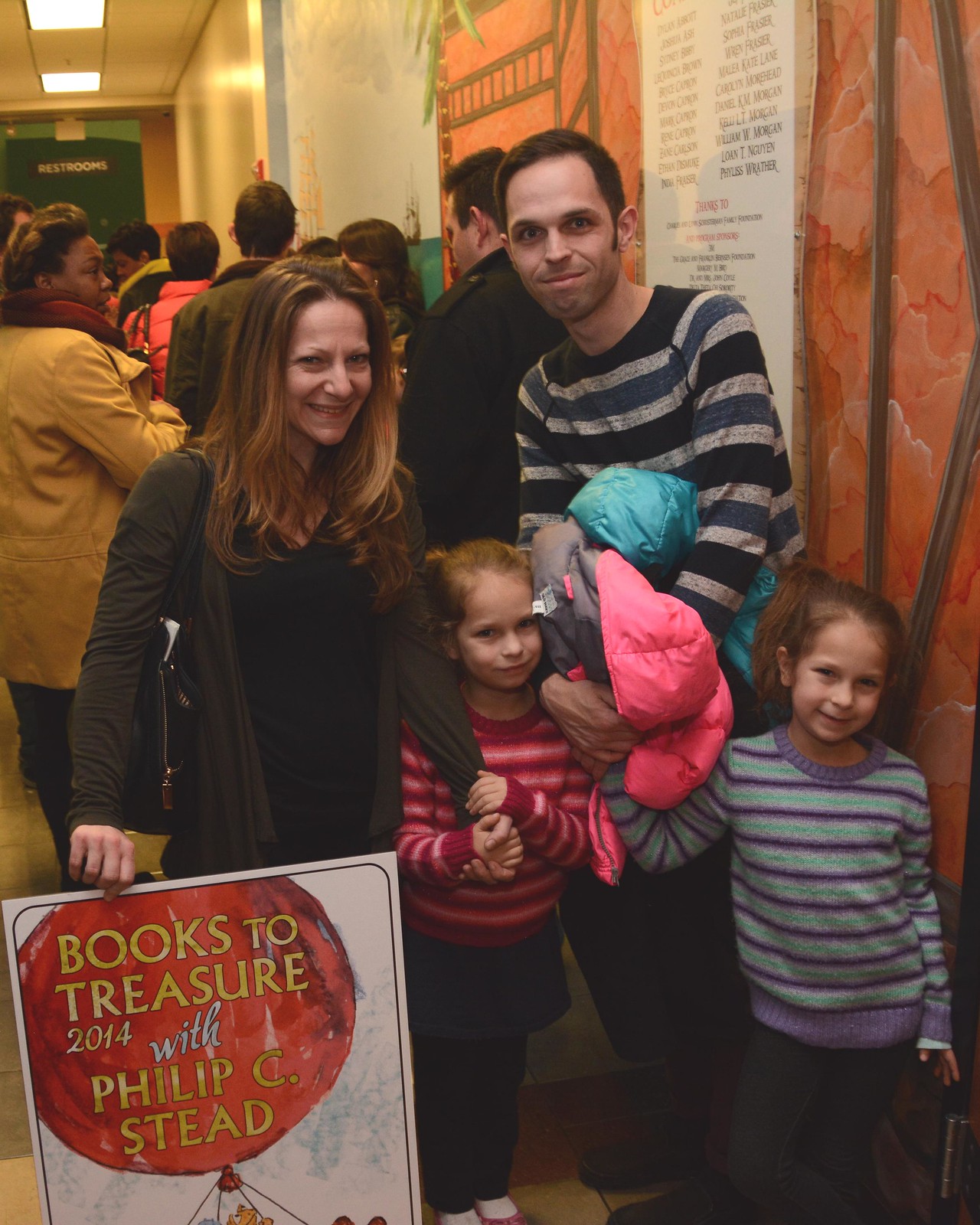In this digital photograph, a happy family is posing in a hallway filled with people. At the forefront are a man, a woman, and two young girls, all wearing striped sweaters—the man's in blue and gray, one girl’s in pink and red, and the other girl’s in blue and purple. The man is holding a blue coat and a pink coat, likely belonging to the girls, while also clasping one girl’s hand. The woman, dressed in a green coat and black shirt, is holding a sign that reads "Books to Treasure 2014 with Philip C. Stead." Both girls are smiling and holding their parents' hands. Behind the family, the hallway buzzes with other people going about their activities, adding a lively backdrop to the scene. Red, yellow, white, purple, pink, and blue colors punctuate the image, contributing to its vibrant and warm atmosphere. To the left of the family, a large red balloon hovers near the top of the sign, suggesting the event is related to books and learning, possibly at a school.